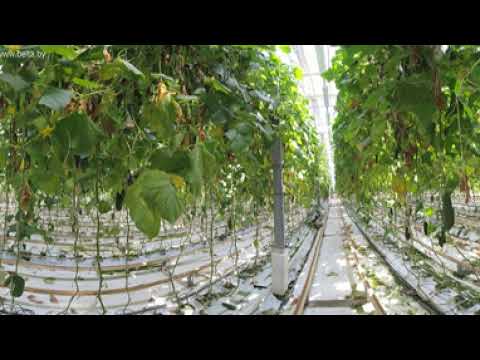The photograph depicts the interior of a large, industrial greenhouse. Within the greenhouse, rows upon rows of green, viney plants stretch from the left to the right, their leafy growths thriving under the ample sunlight that filters through the glass-paneled roof. The bright, natural lighting suggests that the image was taken during the day. The floor appears to be covered with a white material, possibly plastic, which presumably shields the underlying dirt. Numerous metal or steel beams rise from the ground to the ceiling, providing structural support. Although the image is somewhat blurry, the organized layout and the pristine conditions emphasize this as a highly controlled agricultural environment aimed at possibly growing food or other crops. There are no visible fruits or berries on the plants, nor are there any people, vehicles, or written markings, reinforcing the focus on the greenery and the bright, airy atmosphere of the greenhouse.